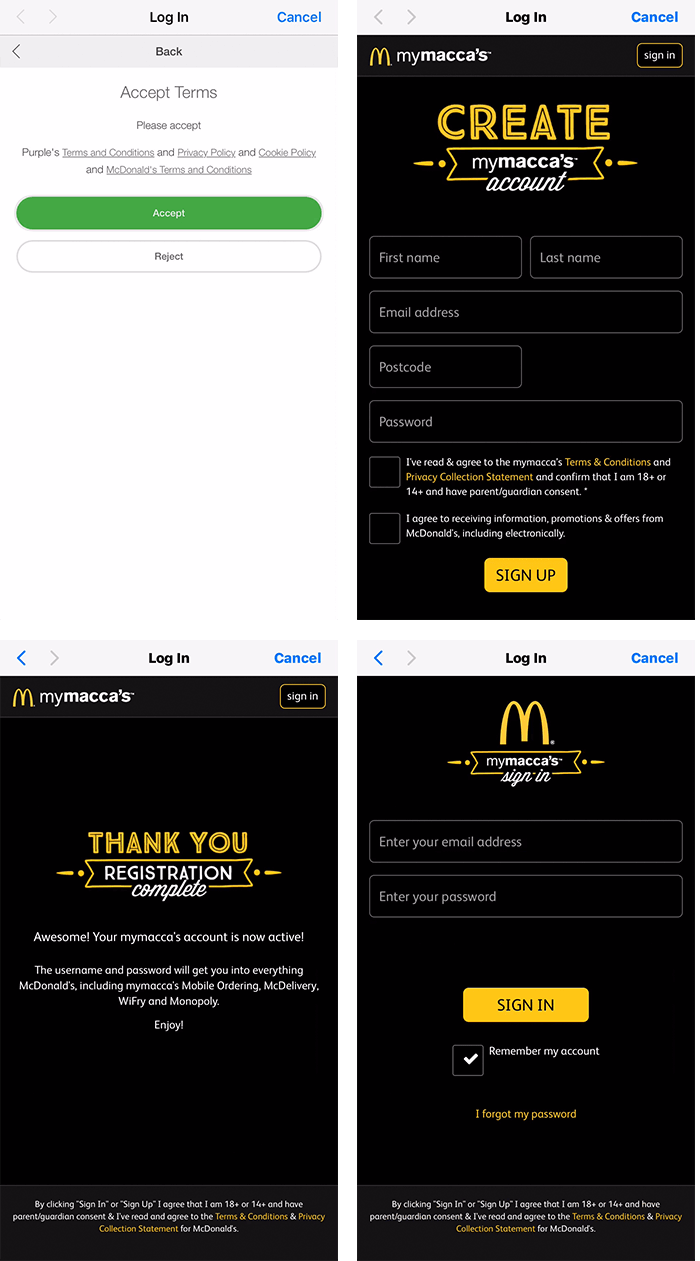The image consists of four screenshots arranged in a grid format, each showcasing a different stage of the MyMACA's account setup and login process:

1. **Top Left Corner: Accept Terms Screen**
   - The screen prompts the user to accept Purple's Terms and Conditions and Privacy Policy.
   - A green "Accept" button and a white "Reject" button are displayed at the bottom.

2. **Top Right Corner: Create Account Screen**
   - This screen is labeled "Create MyMACA's Account."
   - There are text boxes for entering the first name, last name, email address, postcode, and password.
   - Beneath the text boxes, there is a yellow "Sign Up" button and two checkboxes with very small text.

3. **Bottom Left Corner: Registration Complete Screen**
   - The screen displays a message thanking the user and confirming the registration is complete.
   - It states that the user's MyMACA's account is now active and that their username and password will grant access to various McDonald's services, including MyMACA's mobile ordering, McDelivery, Wi-Fi, and Monopoly.

4. **Bottom Right Corner: Sign In Screen**
   - The screen is labeled "MyMACA's Sign In."
   - There are two text boxes: one for the email address and one for the password.
   - Below the text boxes, there is a yellow "Sign In" button.
   - A checkbox labeled "Remember my account" is also present.

Overall, the image captures the step-by-step process from accepting terms and creating an account to successful registration and logging in to the MyMACA's platform.